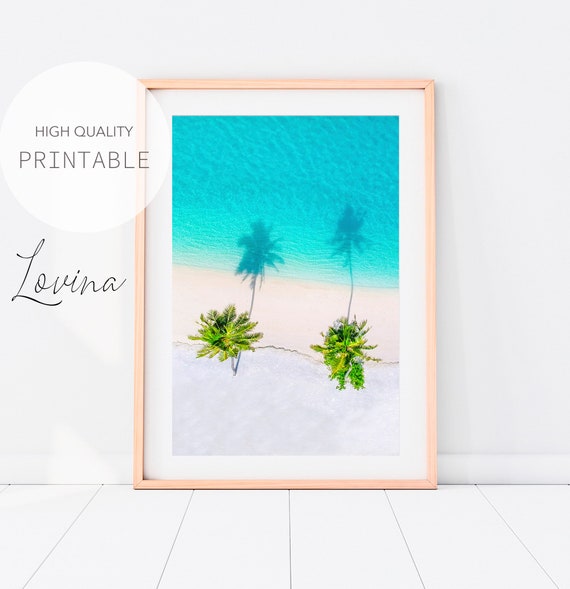This photograph captures a vibrant, tropical-themed print encased in a distinctive pink frame. The print itself showcases an aerial view of two green palm trees casting shadows over the cream-colored sand and turquoise-blue waters, reminiscent of a tropical paradise. The frame, which features a white border, is propped up against a pristine white wall. Beneath the frame, the floor is composed of large wooden boards, painted white, which enhance the overall bright and clean aesthetic of the scene. On the upper left corner of the image, a white circle bubble contains the text "high-quality printable," and just below this bubble, in elegant black cursive, is the word "Lovina." This suggests that the image could be a digital print available for high-quality reproduction.